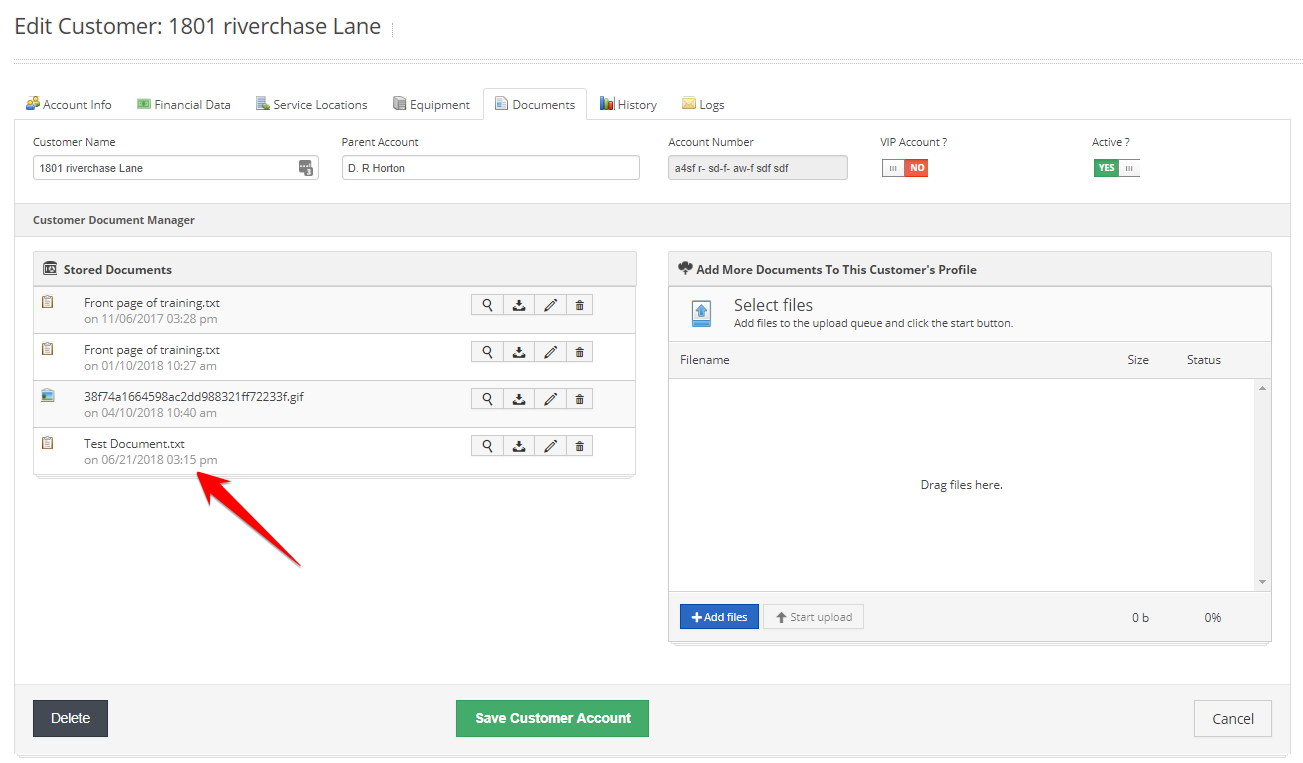Screenshot of an interface titled "Edit Customer 1801 Riverchase Lane," displaying the operational details of a specific customer account. The interface omits the name of the customer, focusing instead on the address "1801 Riverchase Lane." The top menu features tabs labeled: Account Number, Financial Data, Service Locations, Equipment, Documents, History, and Logs. The "Documents" tab is currently active.

Under "Customer Name," the address "1801 Riverchase Lane" is repeated. Further down, details listed include "Account," "Permit Account," referencing "D.R. Horton," and "Parent Account" again as "D.R. Horton." The status of the account is indicated: it is active but not a VIP account.

Beneath this information lies the "Customer Document Manager," showing several stored documents:
1. "Front Page of Training" dated November 6, 2017
2. Another "Front Page of Training" dated January 10, 2018
3. A document labeled "GIF"
4. A "Test Document"

An option to add more documents is provided with a "Select Files" button, which has not yet been utilized, suggesting ongoing or incomplete work on this customer's account.